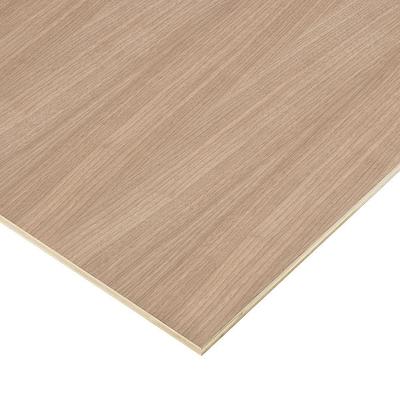This detailed color photograph features a five-sided piece of light to medium brown wood with prominent grain patterns. The piece of wood is positioned diagonally within the frame, creating a dynamic visual effect. The wood extends from the top, descending halfway down the left side and only halfway down the right before angling towards the bottom right middle and then up towards the middle left, forming a unique five-sided shape. The background of the photograph is stark white, emphasizing the rich, varied tones of the wood. The grain flows from the top, sweeping down from right to left, showcasing varying shades of brown. This photograph captures the natural texture and intricate patterns of the wood, with no additional elements such as writing, animals, people, buildings, or mechanical objects present, ensuring the focus remains solely on the wooden piece.